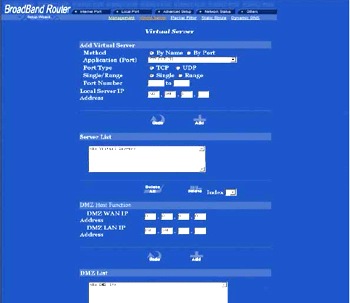The image depicts a user interface of a Broadband Router with a structured layout. At the top, a series of dark blue tabs provide various navigational options. Just below, a lighter blue section contains additional selectable headings, one of which is highlighted in orange, indicating it is the current selection.

Centering on the main screen with a blue background, the primary heading reads "Virtual Server." Below this, there is a banner for adding a virtual server, allowing the user to specify details such as the server name, port, and whether the type is UDP or TCP. Various settings for the IP address can also be configured here.

Directly beneath this, another section titled "Server List" features an editable box where users can list server names. Following this, a panel entitled "DMI MAC Function" includes fields for entering a WAN IP address and a DMZ LAN IP address.

Lastly, at the bottom, the "DMZ List" section provides another editable box, similar to the server list, for listing servers within the DMZ. All these elements are set against a uniform blue background, creating a cohesive visual framework.